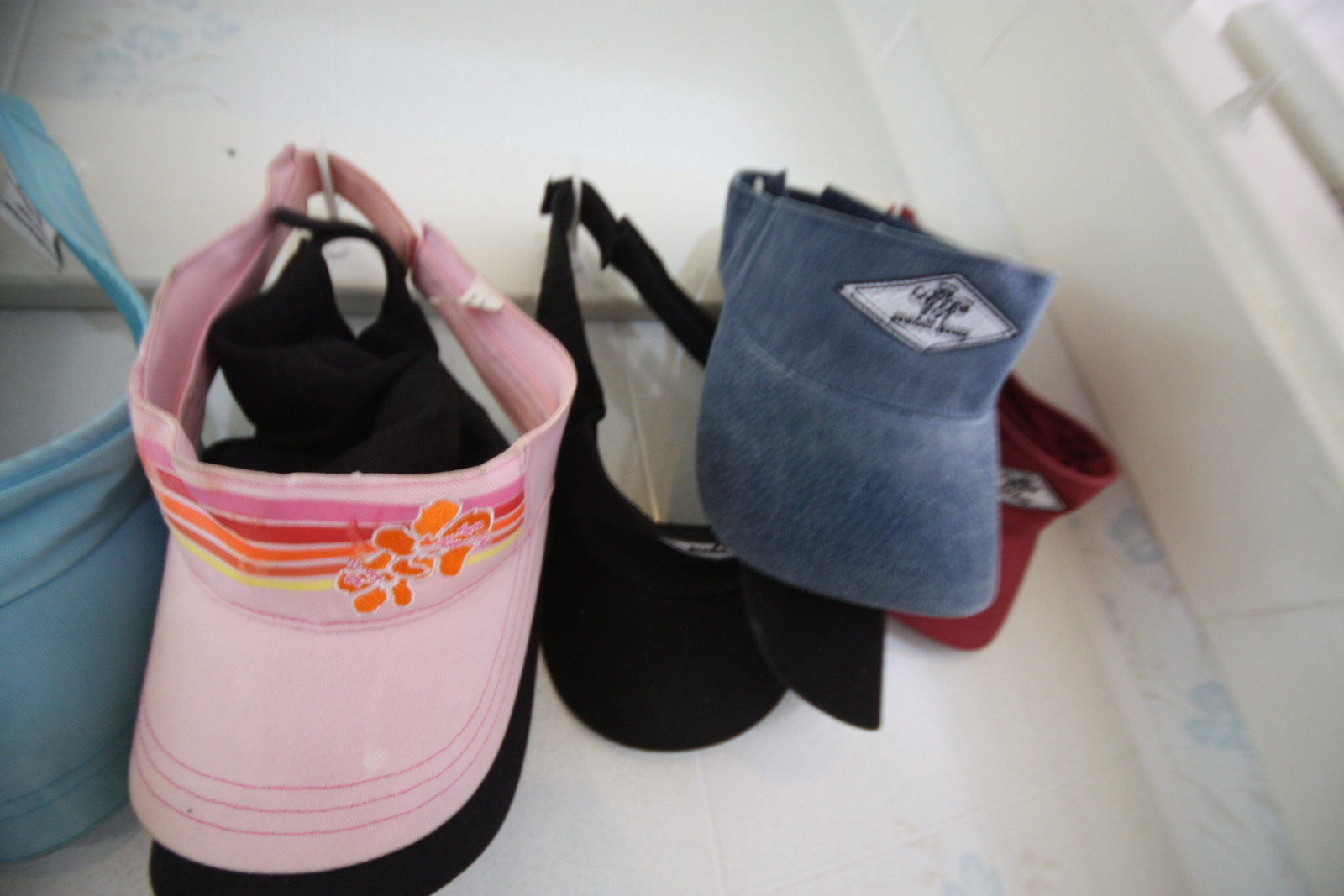The image depicts a neatly arranged display of various sun visor caps hanging on white hooks against a white tiled wall. The caps are suspended from a small, white plank that is securely fastened to the wall, near a white door. In total, there are seven visors in a variety of colors: red, light blue, dark blue, three black, and one pink. The pink visor stands out with its large, colorful flower design and striped pattern on the brim. Both the red visor and the dark blue visor feature a white logo on the front. The other visors - two black ones and a light blue one - are solid in color. The setup appears to be organized and well-maintained, with each visor hanging from its own individual white peg on the board.